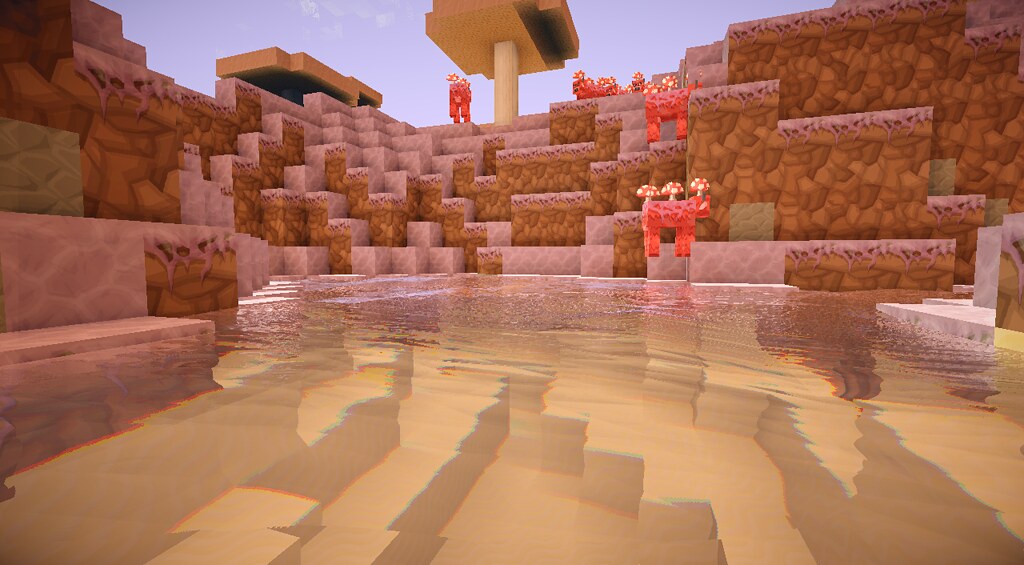This still from a video game features an intricate scene centered around a pool of water in the foreground and middle ground. The environment is dominated by a series of irregular, stair-stepped walls on the left, center, and right, constructed with textured brownish-tan stone. These walls create a visually interesting, multi-layered backdrop. Scattered throughout the scene are various blocky creatures, each adorned with three mushroom-like growths. The creatures exhibit a pink hue with red splotches and vary in their positions and orientations; some are floating, potentially aided by the mushrooms, while others stand atop the walls, adding a dynamic and somewhat mystical element to the landscape.